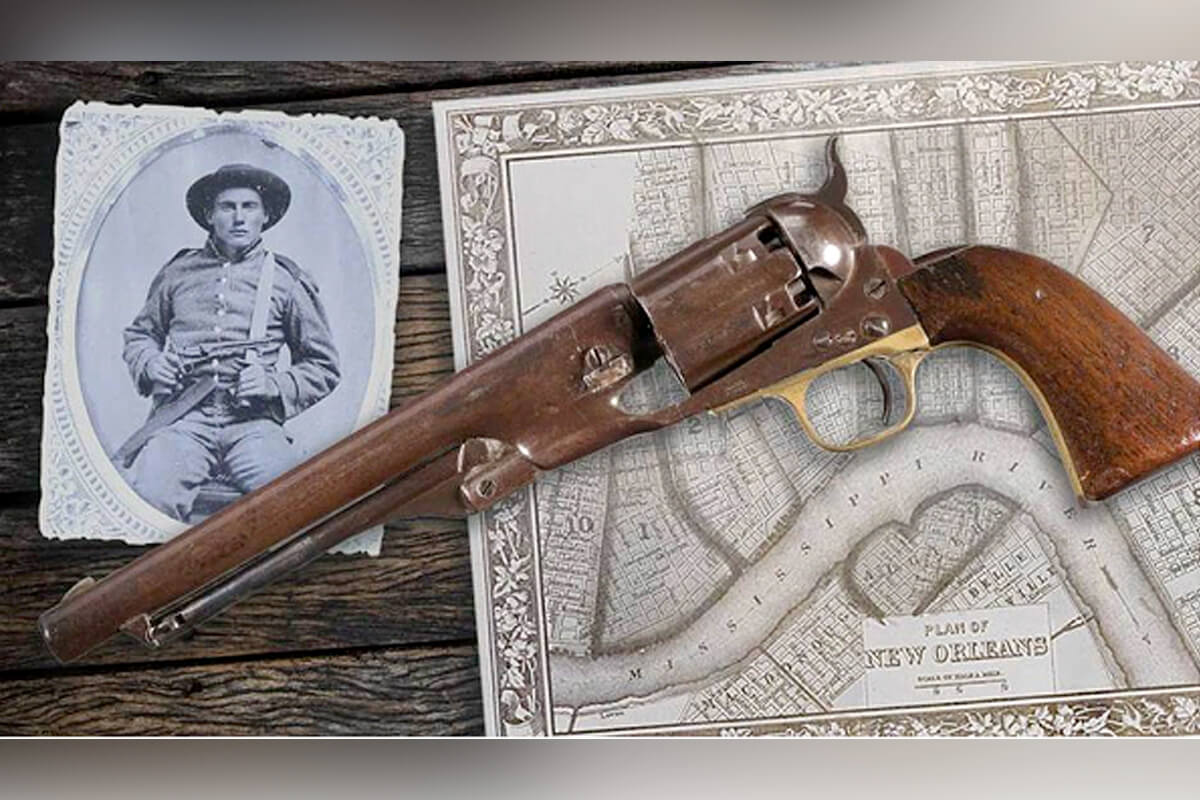The horizontally rectangular, professionally staged photograph features a vintage handgun and historic imagery against an aged wooden backdrop, composed under artificial indoor lighting. Central to the image is a vertically positioned, weathered wood plank with a gray border at the top and bottom. On the left side of this plank, there is a black-and-white photograph of a Civil War-era soldier dressed in period attire, including suspenders and a hat. The soldier is holding a pistol across his body, which closely resembles the actual gun laid out in the scene.

The gun, positioned diagonally with its wooden grip towards the top left, has a barrel displaying signs of rust and a trigger area with a gold hue. The handgun rests on a wooden surface. Beneath the gun, a map of New Orleans can be discerned, characterized by a white background and brown ink. The soldier's framed image sits adjacent to the gun, its white frame standing out against the rustic backdrop.

The composition of the photograph uses a palette of browns, golds, whites, grays, and dark browns, creating an evocative and aged aesthetic. The scene as a whole is captured from a top-down perspective, visually connecting the antique firearm and the historical context through the man's photograph and the map below. The text on the map appears to read "Play o7" alongside the location "New Orleans," though its exact significance remains unclear.